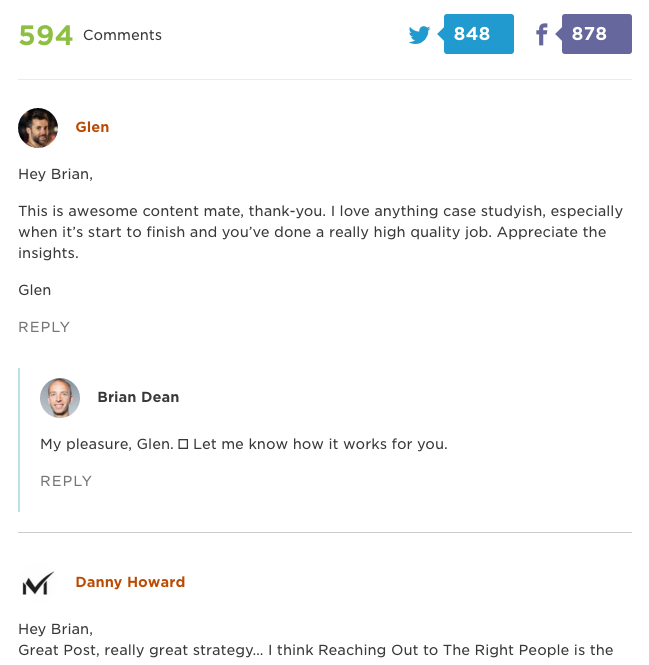This image appears to be a screenshot of the comments section on a website. At the top, social media buttons for Twitter and Facebook are visible, suggesting an option to share content. The header also shows '594 comments' highlighted in green, indicating the current number of comments, which updates dynamically as new comments are added.

The visible comments are as follows:

1. **Glenn**:
   - **Comment**: "Hey Brian, this is awesome content, mate. Thank you. I love anything case study-ish, especially when it's start to finish and you've done a really high-quality job. Appreciate the insights. Glenn."
   - **Avatar**: A headshot image.

2. **Brian Dean** (presumably the author):
   - **Comment**: "My pleasure, Glenn. Let me know how it works for you."
   - **Avatar**: A headshot image.

3. **Danny Howard**:
   - **Comment**: "Hey Brian, great post, really great strategy. I think reaching out to the right people, THAT'S..." (the comment is clipped at this point).
   - **Avatar**: A unique icon resembling a checkmark between two vertical lines.

The commenters' avatars add a personal touch, with Glenn and Brian using headshot photos and Danny Howard using a distinctive icon, which may imply verification or a custom graphic. This detailed interaction highlights a positive engagement between the content creator and the audience, fostering a sense of community and appreciation for high-quality content.